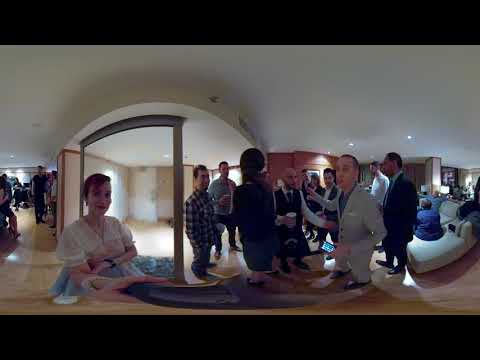The image is a color indoor photograph captured with a 360-degree panoramic lens, resulting in a slightly warped perspective and bounded by black bars at the top and bottom, giving it a cinematic feel. The setting is a large room with white ceilings featuring recessed lights and a mix of tan and brown walls, including a red accent wall adorned with a framed piece of artwork. The floor is a reflective yellow tile, contrasting with some sections of brown hardwood. 

The space is bustling with people engaging in what appears to be a social gathering or casual office meeting. The crowd is diverse, consisting of mostly white individuals with at least one Asian person. Most faces are a bit blurry, but some individuals stand out prominently. To the left, a woman with red hair and wearing a white top is reaching out, possibly adjusting the camera. A man in a gray suit stands to the right, looking towards the camera, with another man in a black suit behind him. Another man, dressed in a black vest, white shirt, and blue tie, holds a compass and faces the camera as well.

Towards the center-right, a grey couch seats multiple people, while another white couch is positioned further back. Lamps are lit in the distance, and glass partitions create semi-enclosed areas with visible doorways and windows. People are distributed throughout the room, standing, sitting, and talking in different clusters, contributing to the dynamic and busy atmosphere.